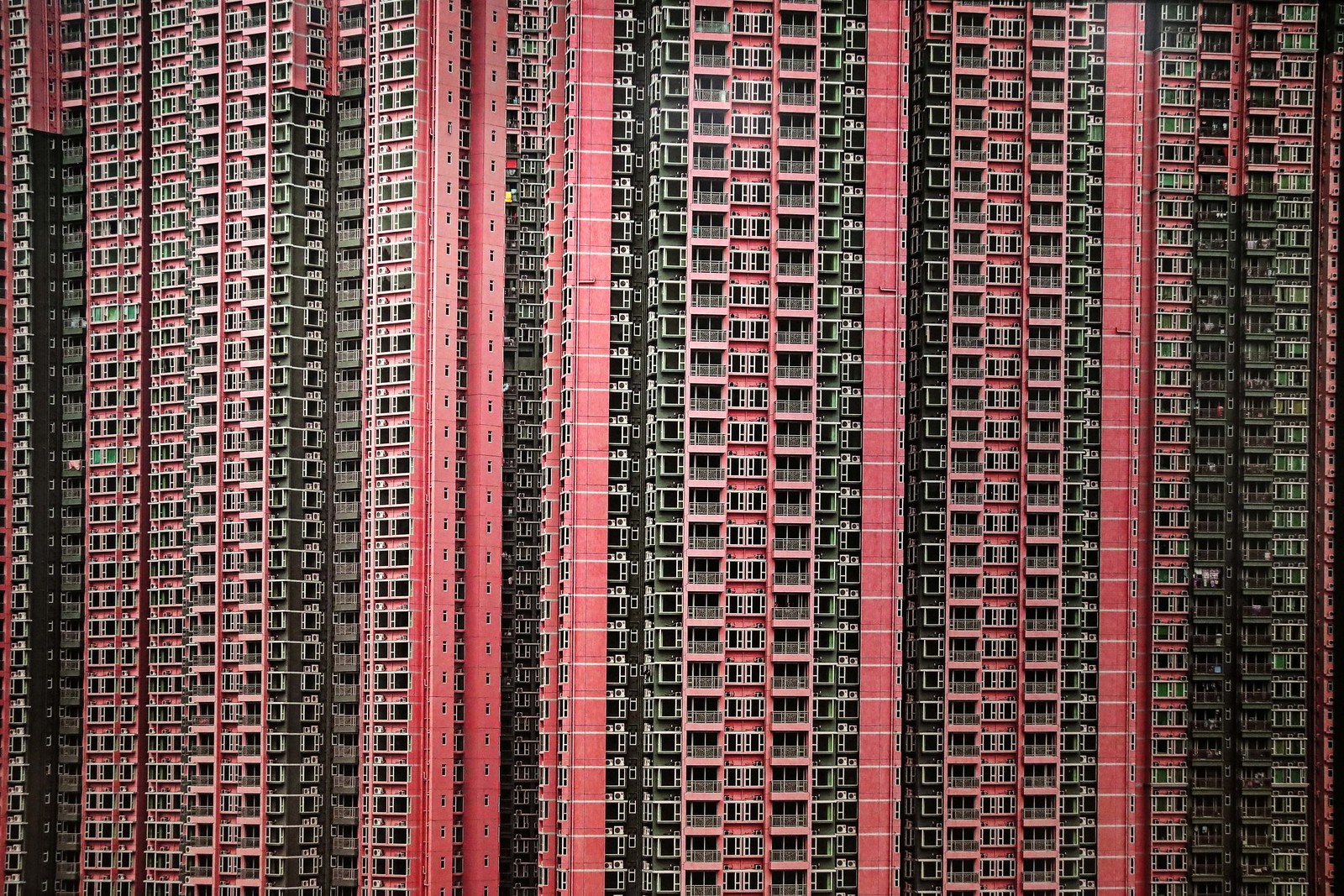The image depicts a towering residential skyscraper, ascending at least 20 stories high, although the top and bottom are not visible, suggesting an even greater height. The façade is characterized by a repetitive pattern of apartment windows, patios, and contrasting colors dominated by light red, pink, and black. The building's exterior features a series of vertical stripes: black, pink with black windows, sections with white patios, and solid pink bars with narrow openings. The balconies, each accompanied by adjacent windows, appear lifeless, with no signs of inhabitants or interior lights. The columns of red bricks interspersed between apartments suggest locations for elevator shafts, essential for accessing the numerous high-density residential units. The overwhelming number and uniformity of windows create a densely packed, imposing structure, likely reminiscent of urban residential buildings in highly populated cities such as those found in China or Japan.